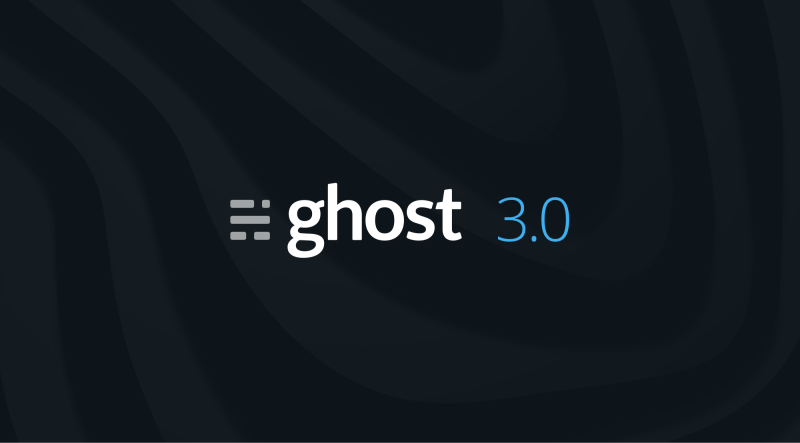The image features a predominantly black, rectangular background, wider than it is tall, adorned with faint, thick, wavy gray lines that transition from thin to thick and swirl in different directions, creating subtle vertical and horizontal patterns. In the center, the word "ghost" appears in bold, lowercase white letters, followed by a space and then "3.0" in a lighter blue, thin font. To the left of "ghost," there is an icon consisting of three horizontal gray lines: the top line is medium gray and partially split on the right side with a small gray square beside it, the middle line is completely solid, and the bottom line is once again split, but this time in the middle, with a black space interrupting it.